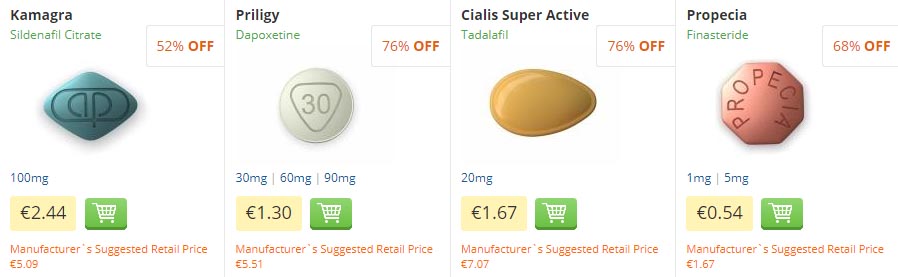A screenshot of a website displaying various pill products for sale, each presented in a distinct section separated by thin gray lines on a white background. The four products include:

1. **KAMAGRA**: 
   - **Active Ingredient**: Sildenafil Citrate (in green font)
   - **Discount**: 52% off (displayed in an orange and white box)
   - **Pill Image**: Teal pill with letter markings
   - **Dosage**: 100 milligrams (in blue font)
   - **Price**: 2.44 pounds (in black font inside a yellow box)
   - **Additional Info**: Manufacturer's suggested retail price of 5.09 pounds (in green and orange font)
   - **Cart Icon**: Green and white

2. **Priligy**:
   - **Active Ingredient**: Dapoxetine (in green font)
   - **Discount**: 76% off (displayed in orange)
   - **Pill Image**: Round white pill with the number "30" on it
   - **Dosage Options**: 30, 60, 90 milligrams (in blue font)
   - **Price**: 1.30 pounds (in black font inside a yellow box)
   - **Additional Info**: Manufacturer's suggested retail price of 5.51 pounds (in orange font)
   - **Cart Icon**: Green and white

3. **Cialis Superactive**:
   - **Active Ingredient**: Tadalafil (in green font)
   - **Discount**: 76% off (displayed in orange)
   - **Pill Image**: Tear-drop shaped, gold-colored pill
   - **Dosage**: 20 milligrams (in blue font)
   - **Price**: 1.67 pounds (in black font inside a yellow box)
   - **Additional Info**: Manufacturer's suggested retail price of 7.07 pounds (in orange font)
   - **Cart Icon**: Green and white

4. **Propecia**:
   - **Active Ingredient**: Finasteride (in green font)
   - **Discount**: 68% off (displayed in orange)
   - **Pill Image**: Salmon-colored pill stamped with 'Propecia' in a circular pattern
   - **Dosage Options**: 1 milligram, 5 milligrams (in blue font)
   - **Price**: 0.54 pounds (in black font inside a yellow box)
   - **Additional Info**: Manufacturer's suggested retail price of 1.67 pounds (in orange font)
   - **Cart Icon**: Green and white